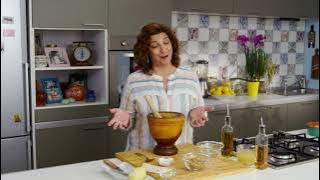In the screenshot of a video, a woman is standing in a kitchen behind a counter, seemingly engaged in a TV cooking class. Her dark brown, shoulder-length curly hair frames her calm, contemplative expression with her eyes slightly closed and hands extended in front of her, palms up as if deep in thought. She wears a white blouse adorned with gray and yellow vertical stripes.

In the foreground, a prominent wooden-colored chopping block hosts a large, dark brown mortar and pestle accompanied by light yellow implements. Surrounding the setup are glass bottles containing various liquids, hinting at cooking ingredients. To the right of the counter, a black stove top integrated into the kitchen island is visible. 

The background showcases kitchen elements, including a silver refrigerator on the far left, a pair of shelves amidst greenish-gray cabinets displaying a white clock, pictures, and books. A tall bunch of purple lilies and bowls of fruit also embellish the shelves. The back wall features a checkered pattern of white and black tiles, and to the far right, a sink can be seen. The scene captures a harmonious blend of culinary activity and kitchen decor, providing a detailed, inviting glimpse into the woman's culinary world.